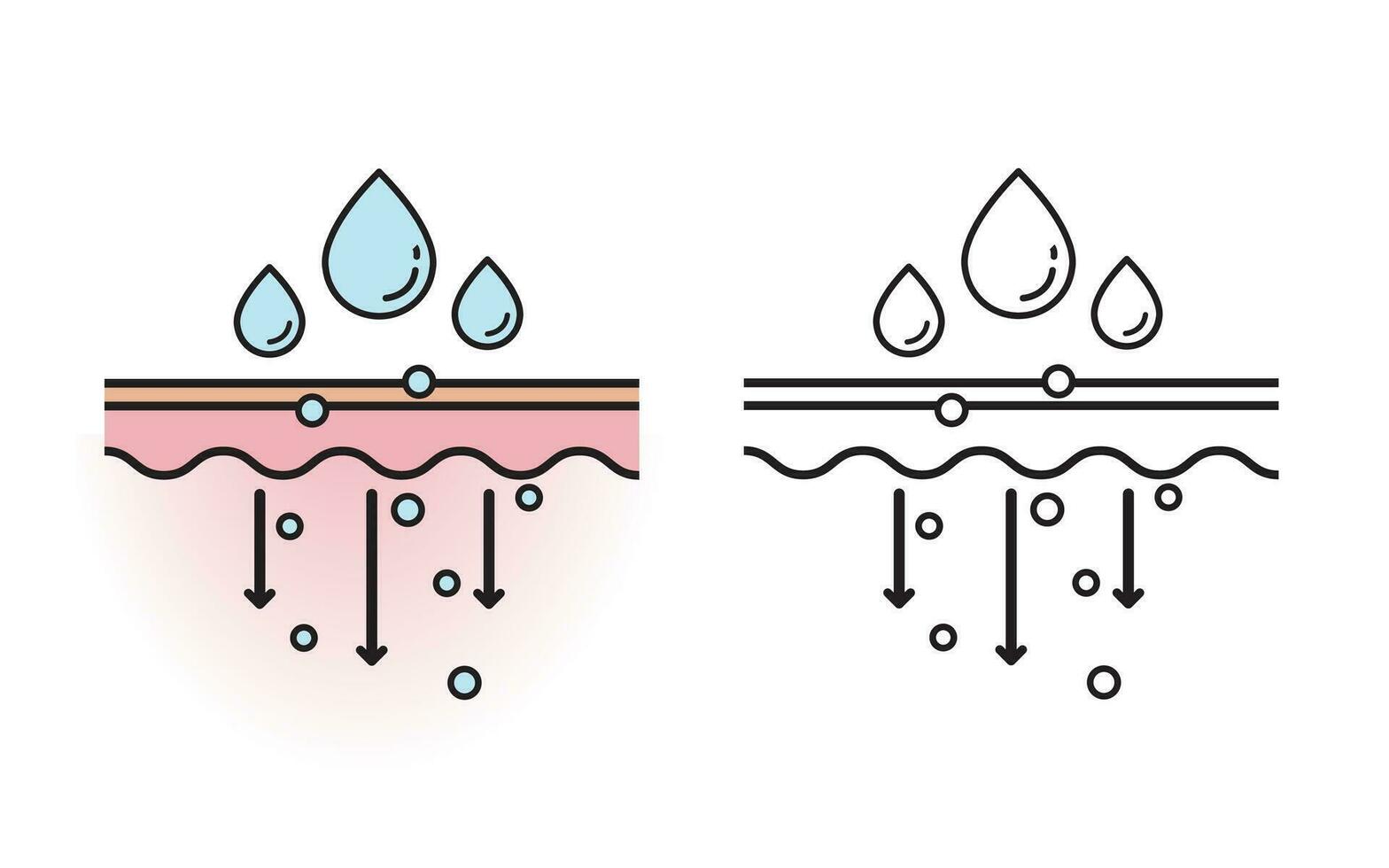This image consists of two mirrored illustrations side by side, highlighting a comparison between color and monochrome depictions. The left side features a color version, whereas the one on the right is rendered in black and white. Both show a sectioned earth profile. The top layer of the ground in the colored version is brown, followed by a thicker, wavy light pink layer beneath. Above this ground section, three light blue water droplets are visible, and three more droplets in the same color are depicted below the surface, along with arrows pointing downward. The corresponding right-hand side image is identical in structure but uses only black and white. Here, the droplets, layers, and arrows are all outlined or filled in with varying shades of black, highlighting the same details but without the use of color.